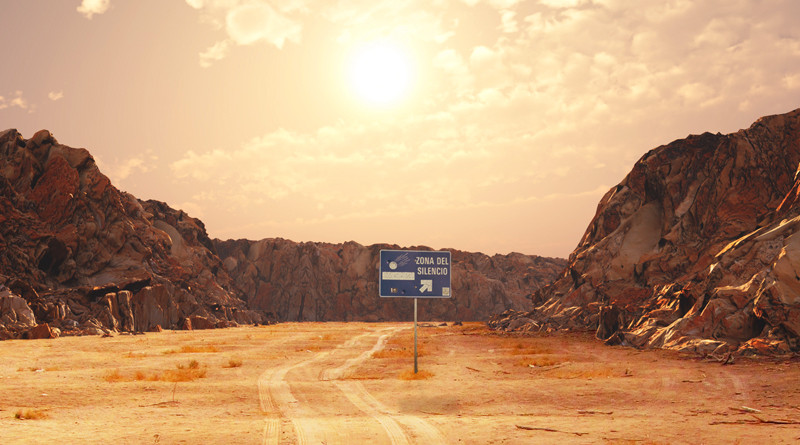The photograph captures an isolated dirt road winding through a desolate desert landscape, marked only by a set of tire tracks meandering through a sandy pass flanked by tall, rugged cliffs. These cliffs, towering approximately the height of three people stacked vertically, are composed of various tan, white, and gray rocks, devoid of any visible vegetation. Scattered beside the tire tracks, sparse patches of dead green and yellow vegetation struggle against the barren expanse. Dominating the scene is a dark blue, rectangular sign mounted on a pole, inscribed with the words "Zona del Silencio" in white text, indicating the mysterious and remote nature of the location. Above, the sky is a hazy gray-orange hue, with white clouds scattered around the centered, brightly shining sun, casting an otherworldly glow over the stark and silent terrain.